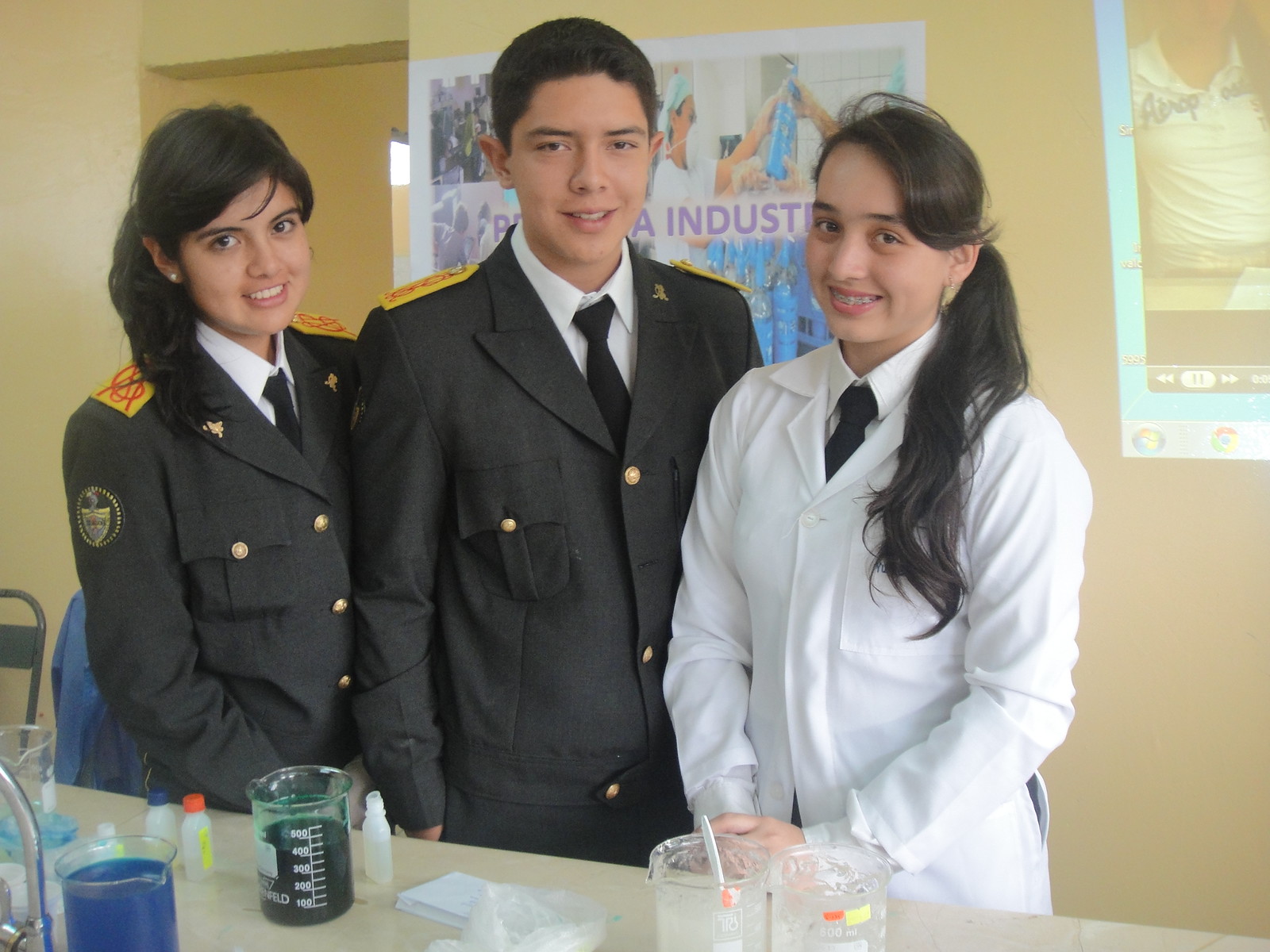This photo captures three young individuals, likely siblings, in a laboratory setting. Two of them are dressed in identical dark military uniforms adorned with gold buttons and yellow shoulder patches, suggesting they might be in the army or navy. The woman on the left has dark hair styled in a ponytail, and the man next to her, also with dark hair, mirrors her appearance and attire, indicating a strong familial resemblance. The third individual, a woman, stands on the right, wearing a white lab coat over a collared shirt and white tie, indicating her role as a scientist or lab assistant. Her dark hair is similarly tied back, with her ponytail draped over her shoulder. They are positioned behind a light beige-to-white countertop, which holds various glass beakers filled with liquids, indicative of their lab environment. The background shows beige walls, and all three are smiling warmly at the camera, suggesting a moment of camaraderie amidst their professional roles.